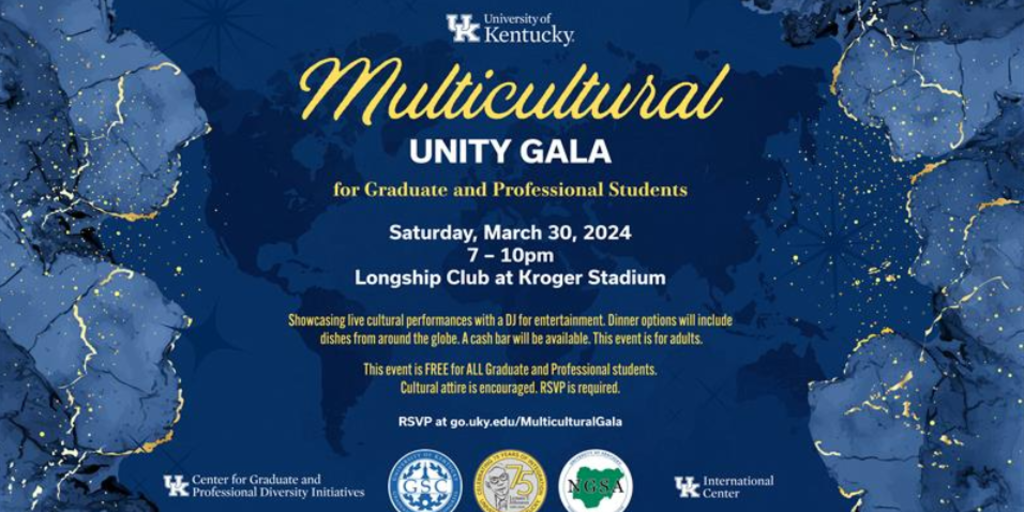The image is an infographic advertisement for the Multicultural Unity Gala at the University of Kentucky. Set against a predominantly blue background, the design features a world map in various shades of blue, embellished with gold trim and golden speckles. The left and right sides of the image display an abstract pattern with blue textures and gold details. The central text, in golden-yellow and white, announces the event details: "Multicultural Unity Gala for Graduate and Professional Students." The gala will take place on Saturday, March 30th, 2024, from 7 to 10 p.m. at the Longship Club in Kroger Stadium. The event will showcase live cultural performances and a DJ for entertainment. Dinner options will feature dishes from around the globe, and a cash bar will be available. This adult-only event is free for all graduate and professional students. Cultural attire is encouraged, and RSVP is required. The infographic is adorned with logos at the bottom, adding a formal touch to the event presentation.